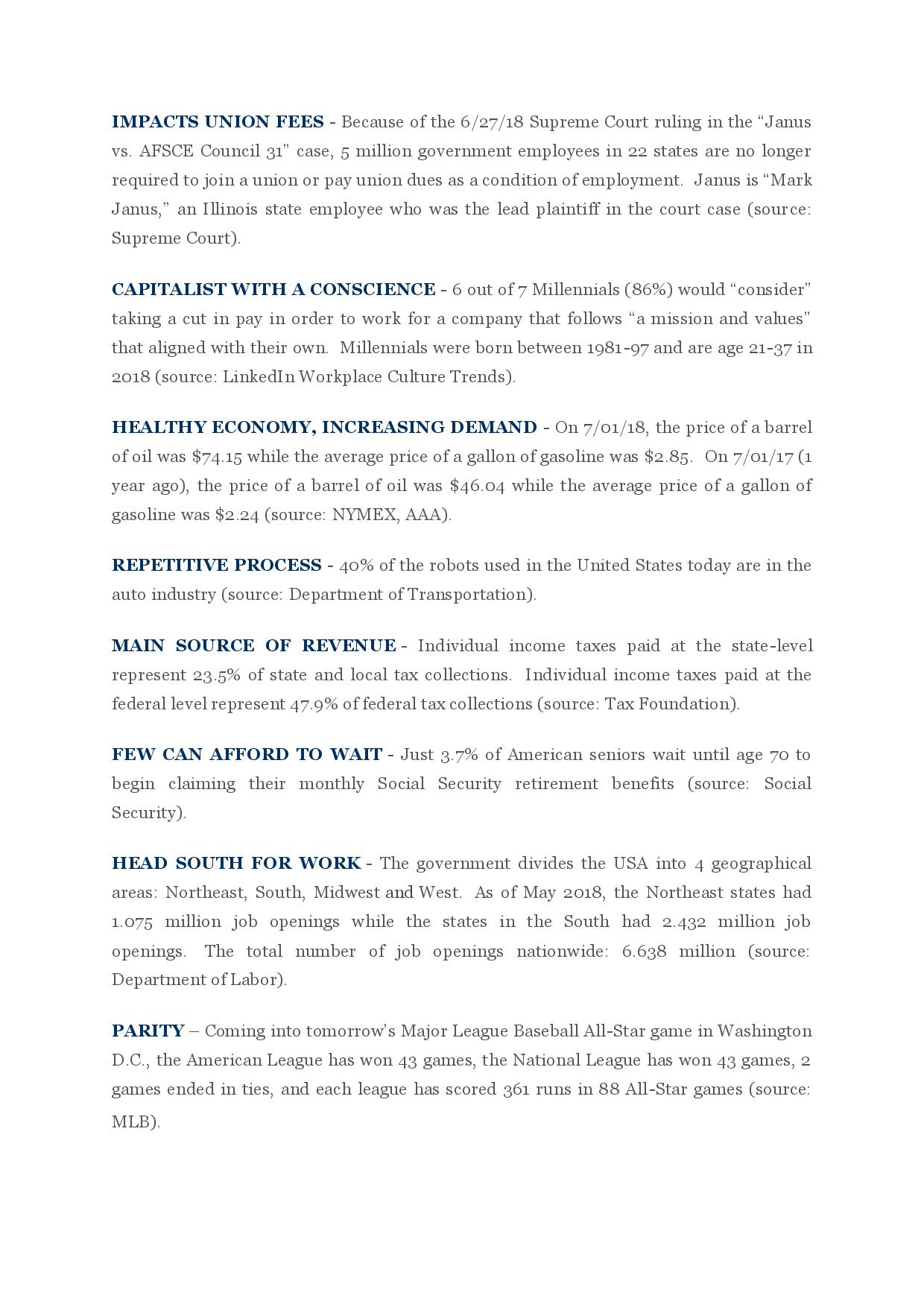Page Display of a Right-Leaning Newsfeed:

This webpage presents multiple news categories, each highlighting significant legal, social, and economic issues. 

1. **Impacts of Supreme Court Ruling on Union Fees**:
   - **Headline**: "Impacts on Union Fees by the Supreme Court's Janus v. AFSCME Council 31 Ruling"
   - **Content**: The Supreme Court's landmark decision in the Janus v. AFSCME Council 31 case (62718) has profound implications for union membership and financing. The ruling declares that approximately 5 million government employees in 22 states are no longer mandated to join a union or pay union dues as a condition of their employment. This case was led by Mark Janus, an Illinois state employee, and has since influenced union policies and rights nationwide. 
   - **Source**: Sourced from the Supreme Court documents.

2. **Millennials' Preference for Value-Driven Employment**:
   - **Headline**: "Capitalists with a Conscience: Millennial Employment Preferences"
   - **Content**: According to a study on LinkedIn Workplace Culture Trends, six out of seven millennials are willing to accept a pay cut to work for companies that share their personal mission and values. The demographic group in focus, millennials, were born between 1981 and 1997 and were aged between 21 to 37 years in 2018. The data highlights the growing importance of corporate social responsibility and alignment of values in employment decisions among younger generations.
   - **Source**: LinkedIn Workplace Culture Trends Report.

Overall, the page resembles a right-leaning newsfeed, structured to present various facts and articles, potentially appealing to an audience with conservative viewpoints.